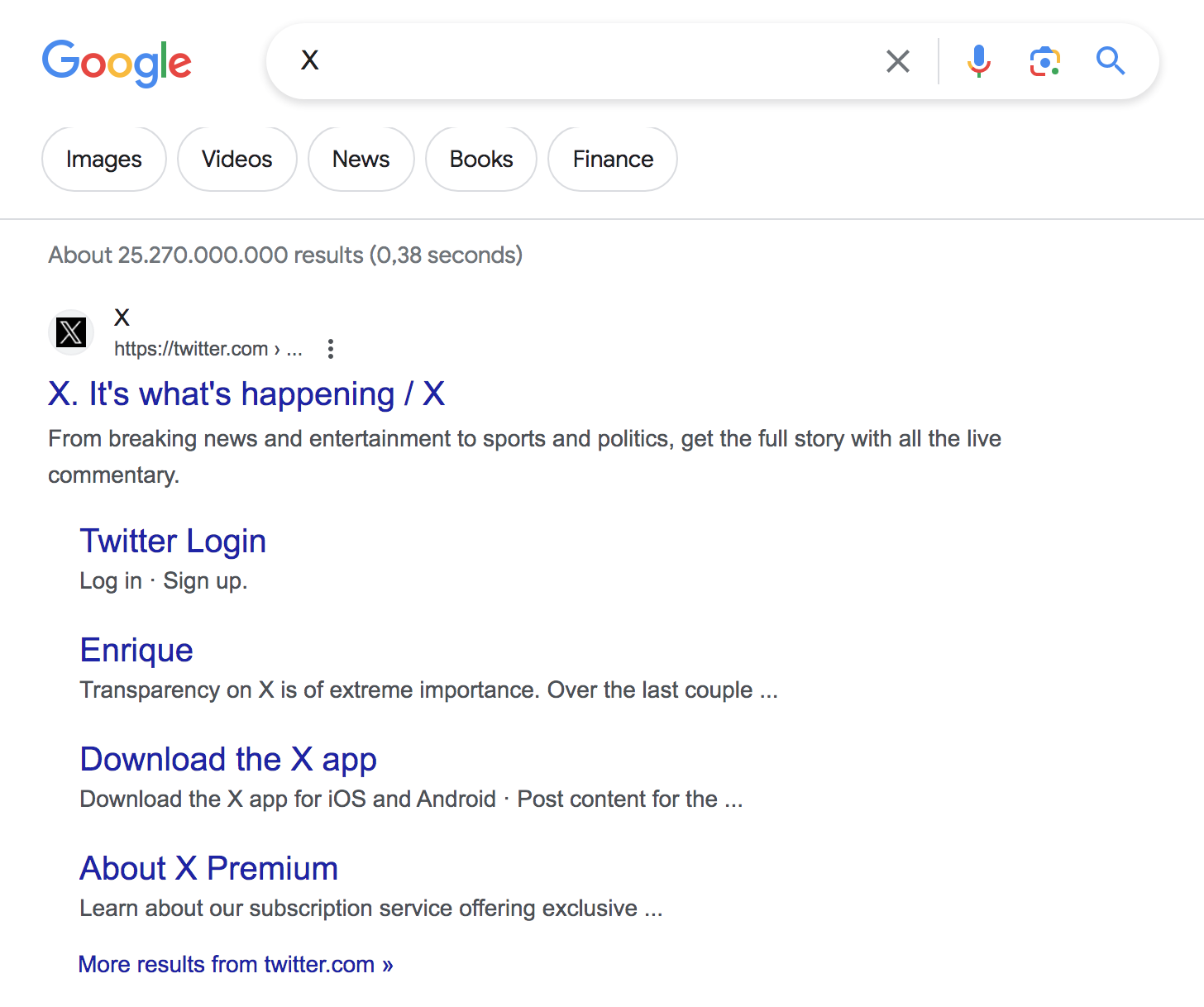The image depicts Google search results. In the upper left-hand corner, the word "Google" is prominently displayed. To its immediate right, after two spaces, is the Google search bar where the query "X" has been entered. Below the search bar, starting from the left, are several buttons labeled "All," "Images," "Videos," "News," "Books," and "Finance."

Beneath these buttons is a subtle gray separator bar. Below the bar, in a smaller font, it states that there are approximately 25,270,000,000 results, fetched in 0.38 seconds.

The top search result is from "X" at twitter.com, accompanied by a tagline that reads, "It’s what's happening." Further details provided in the snippet explain, "From breaking news and entertainment to sports and politics, get the full story with all the live commentary." This introduction provides a brief overview of what X, previously known as Twitter, offers to its users.